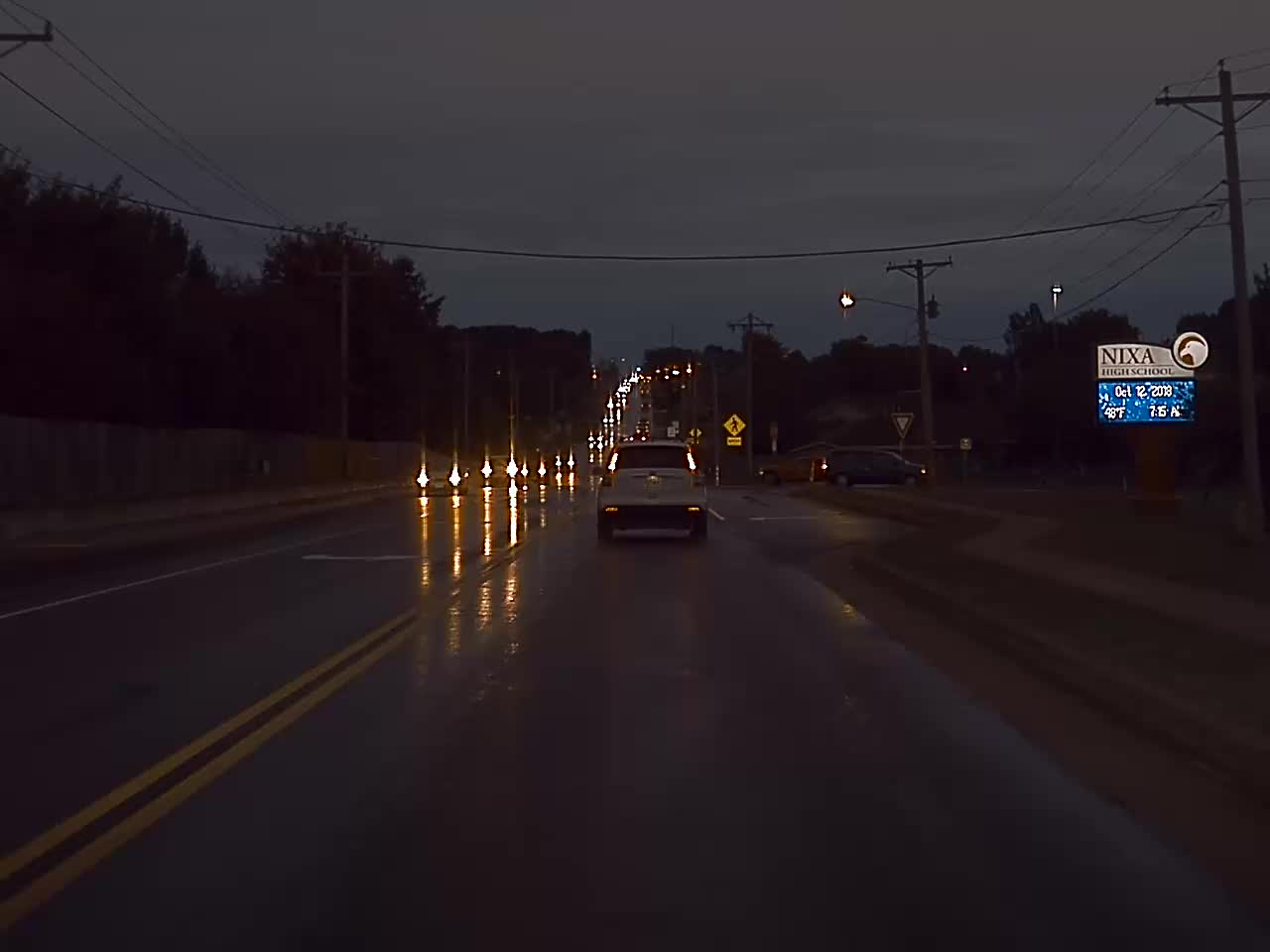This color photograph captures a nighttime scene of a roadway. The central focus is on the road ahead, where a vehicle, likely a truck or lorry, is visible with its taillights glowing faintly in the darkness. The image is quite dim, making it hard to discern specific details of the vehicle. A double yellow line runs along the left side of the road, indicating a no-passing zone, while a stream of oncoming traffic can be seen in the distance, their headlights reflected brightly on the wet road surface.

On the left side of the road, there are trees in the background, a fence, and a small paved area. The right side features a zigzagging path adjacent to the road, along with overhead power lines and an illuminated sign with a gray top and blue bottom, though the text is unreadable. In the far distance, streetlights illuminate the road, and another yellow sign is also visible. Their reflections add a golden hue to the scene, contributing to the overall atmosphere of a silent, darkened roadway.